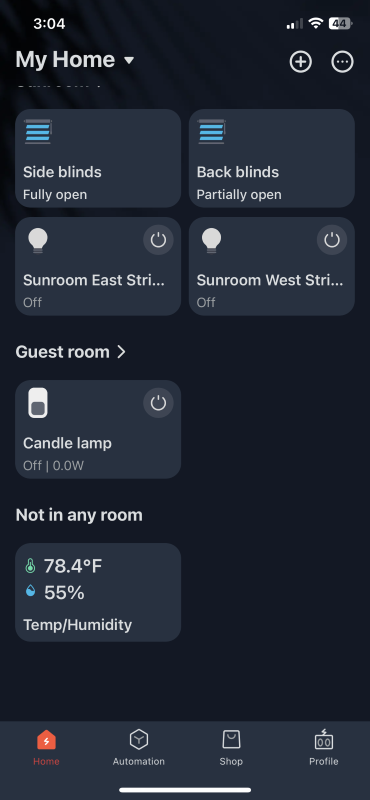Screenshot of a mobile app displaying an IoT (Internet of Things) control menu on a black background with white text. The status bar at the top shows the current time as 3:04, with two bars of service, a fully connected Wi-Fi icon, and a battery level at 44%. 

The 'My Home' tab is active, indicated by a label at the top. On the top right corner, there are two icons: a plus sign and a menu button represented by three vertical dots. 

The main screen details various smart home controls:
- Side Blinds: Fully open
- Back Blinds: Partially open

On the next row:
- Sunroom East Light: Off
- Sunroom West Light: Off

Following that:
- Guest Room Candle Lamp: Off

Additionally, it displays the overall home environment statistics:
- Temperature: 78.4°F
- Humidity: 55%

At the bottom of the screen, there is a standard navigation menu with options: Home, Automation, Shop, and Profile.